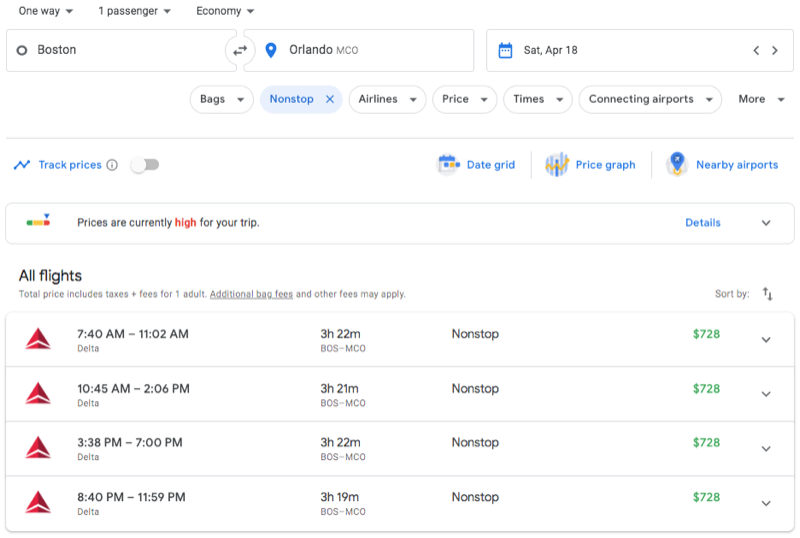A flight booking website displays a search result for flights from Boston to Orlando on Saturday, April 18th. The user has opted to track prices on flights. There are four nonstop flights listed, each priced at $728. 

1. The first flight departs at 7:40 a.m. and arrives at 11:02 a.m., with a flight duration of 3 hours and 22 minutes.
2. The second flight departs at 10:45 a.m. and arrives at 2:06 p.m., taking 3 hours and 21 minutes.
3. The third flight leaves at 3:38 p.m. and lands at 7:00 p.m., lasting 3 hours and 22 minutes.
4. The fourth flight departs at 8:40 p.m. and arrives at 11:59 p.m., with a duration of 3 hours and 19 minutes.

Each option offers the same fare, leaving the decision to book a ticket dependent solely on the preferred departure and arrival times.